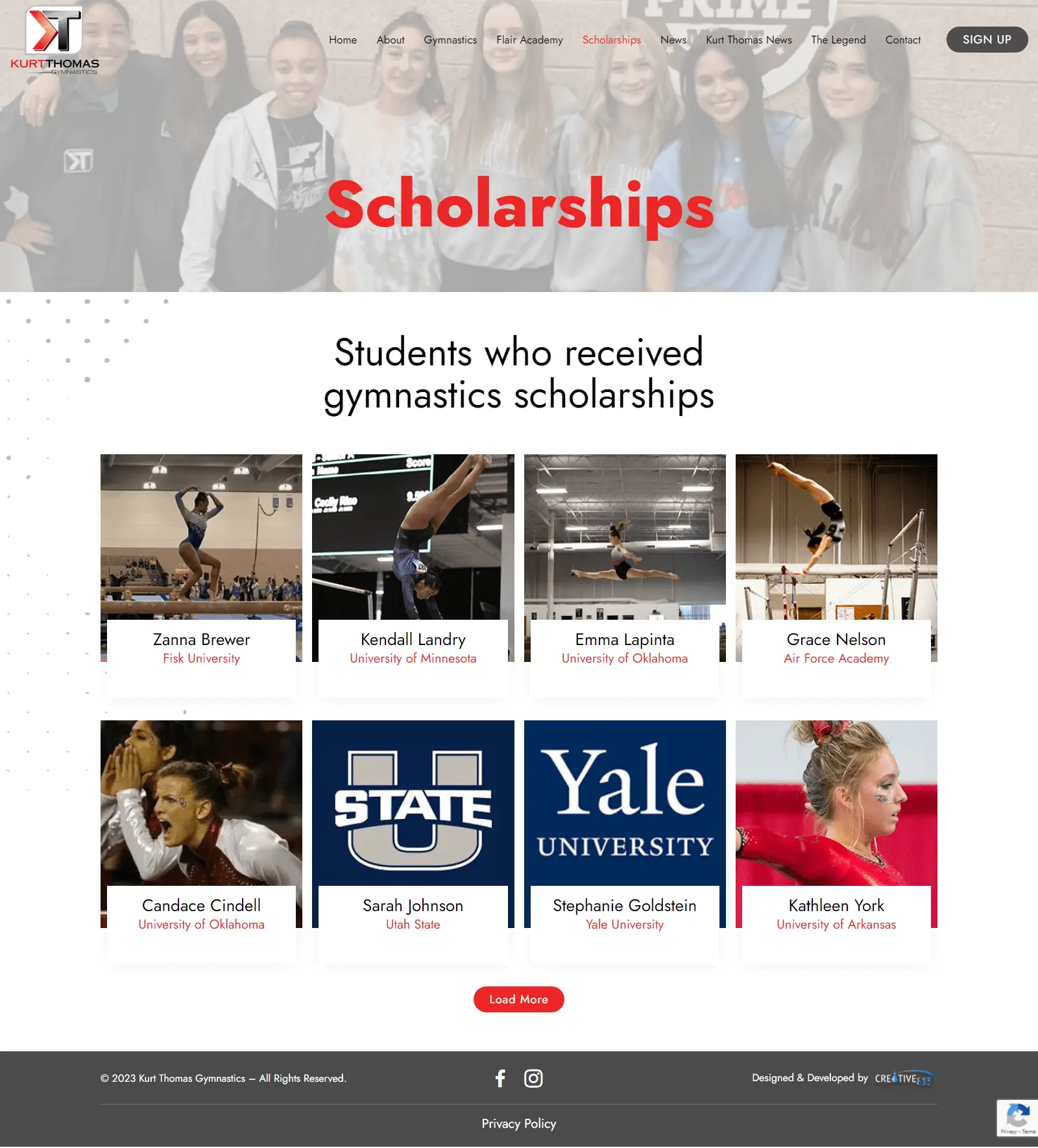The top left corner of the image features the name "Kurt Thomas," with "Kurt" in red and "Thomas" in black, followed by the word "Gymnastics" underneath in black text. The background showcases a photograph of eight high school-aged girls standing together, slightly hazy in appearance. Overlaid on this image, the word "Scholarships" is prominently displayed in red.

At the top of the image, a navigation bar lists the following menu items: Home, About, Gymnastics, Flair Academy, Scholarships, News, Kurt Thomas News, The Legend, Contact, and a black sign-up button with white text. Below the navigation bar, against a white background, the heading "Students Who Received Gymnastic Scholarships" is displayed.

Beneath this heading are two rows of photographs, each containing four images:

**First Row:**
1. **Zaina Brewer** - Fisk University
2. **Kendall Laundrie** - University of Minnesota
3. **Emma Lapintina** (L-A-P-I-N-T-A) - University of Oklahoma
4. **Grace Nelson** - Air Force Academy

**Second Row:**
1. **Candice Sindel** - University of Oklahoma
2. **Sarah Johnston** - Utah State
3. **Stephanie Goldstein** - Yale University
4. **Kathleen York** - University of Arkansas